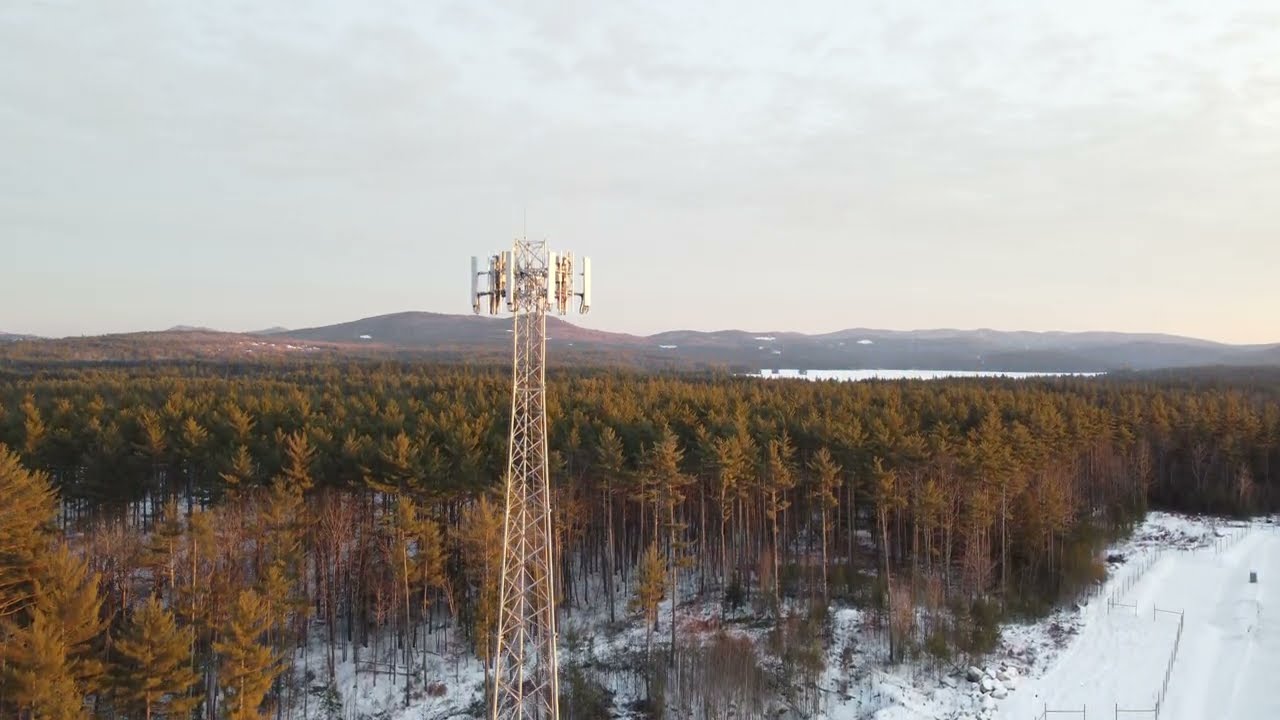The image captures a slightly elevated view of a white cell tower standing tall in the center-left foreground, its top half adorned with various equipment. The tower is surrounded by a wintry scene, where snow covers the lower right-hand corner and patches the ground among a dense forest of green and brown pine trees, their lower halves pruned away. A stretch of fencing can be seen in the snow, suggesting a demarcated private property. Further out, the terrain undulates with low, hilly mountains dusted in snow, extending across the entire background and blending into a brown, greenish, and yellowish mountain range. The sky overhead is a somber light blue-gray, hinting at overcast weather or the onset of dusk, adding a chilly ambiance to the serene, expansive wooded landscape. Beyond the trees lies either a body of water or a snow-covered area, contributing to the wintry feel of the scene.